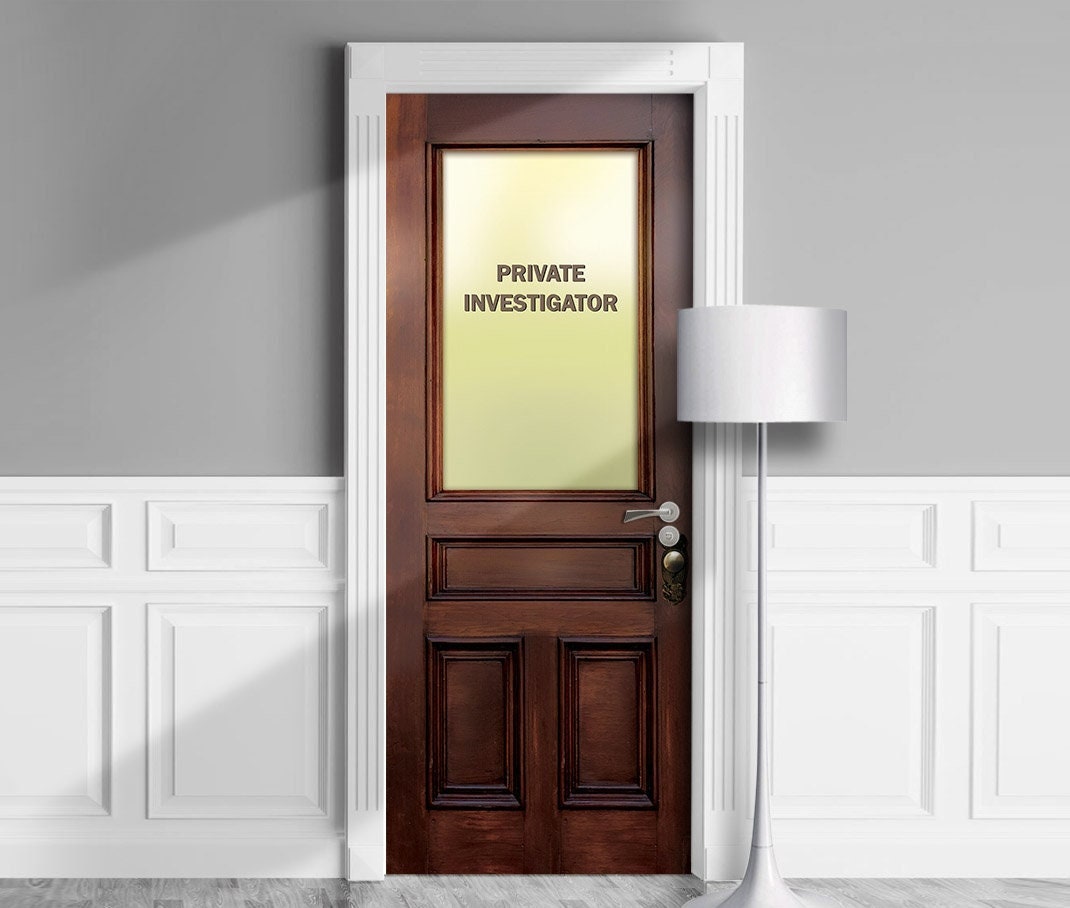The image shows the entrance to a private investigator's office located within a business building. The surrounding walls are grey with white paneling at the bottom. The office door, finished in a wood style, features a central frosted glass panel with the words "Private Investigator" inscribed in dark grey font. Notably, the door is equipped with three separate doorknobs: a circular one, a deadbolt, and a handle at the top. Adjacent to the door, slightly to the right, stands a silver lamp with a matching silver lampshade. The floor outside the office is covered in light grey tiles, adding to the professional ambiance of the setting.